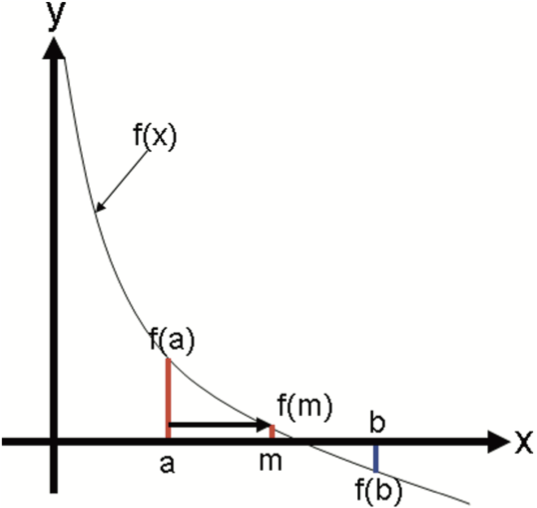The image depicts a detailed diagram of a graphed function with labeled points and arrows. The x-axis and y-axis, both drawn in black, intersect at the origin. The function displays a discontinuity on the y-axis and is illustrated as a thin, curved gray line running from the top left (near the label Y) to the bottom right. Key points A and B on the x-axis correspond to F(A) and F(B) on the y-axis. The midpoint M of A and B maps to F(M) on the y-axis. Key labels include 'F(X)' with an arrow pointing to the line. An upward-pointing tall arrow on the left side bears a lowercase 'y' at the top. A long, thin downward arrow is positioned to the right, accompanied by various arrows pointing rightward. Additional labeled points are depicted: 'F(A)' and 'A' with a tall red line, 'F(B)' with a blue line, and 'F(M)' with a shorter red line, all aligned vertically with their respective x-coordinates. An arrow at the bottom right points rightward towards 'X'. The comprehensive labeling and arrows illustrate various relationships between the x-axis values and their corresponding function values on the y-axis.